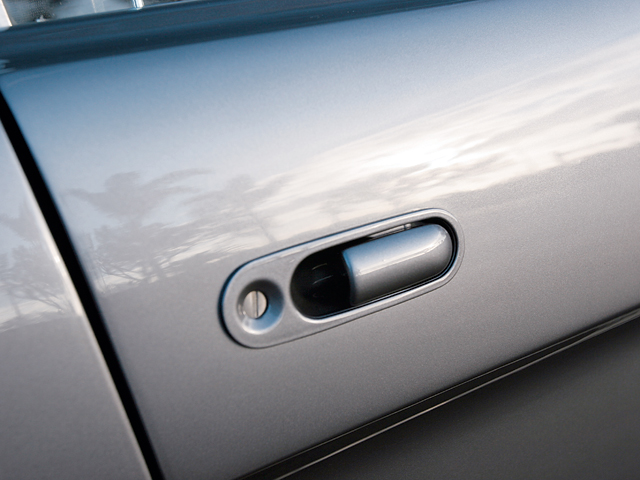This is a very close-up image taken outdoors of a perfectly straight and shiny silver car door and door handle. The door reflects palm trees and a sunset-colored sky, with clouds also visible in the sleek, mirror-like finish. The top part of the door shows darker blue shading from shadows. The detailed door handle in the center has a thin, oval-ish shape with a unique design that includes a black half-oval piece and a silver half-oval that you pull outward to open the door. On the left side of the handle is a circular indent featuring a silver screw, not a keyhole. The door trim includes a rubber piece at the top and silver trim near the bottom, with defined lines indicating where the door would open and close. The door appears slightly tilted in the image, taken at an interesting angle.